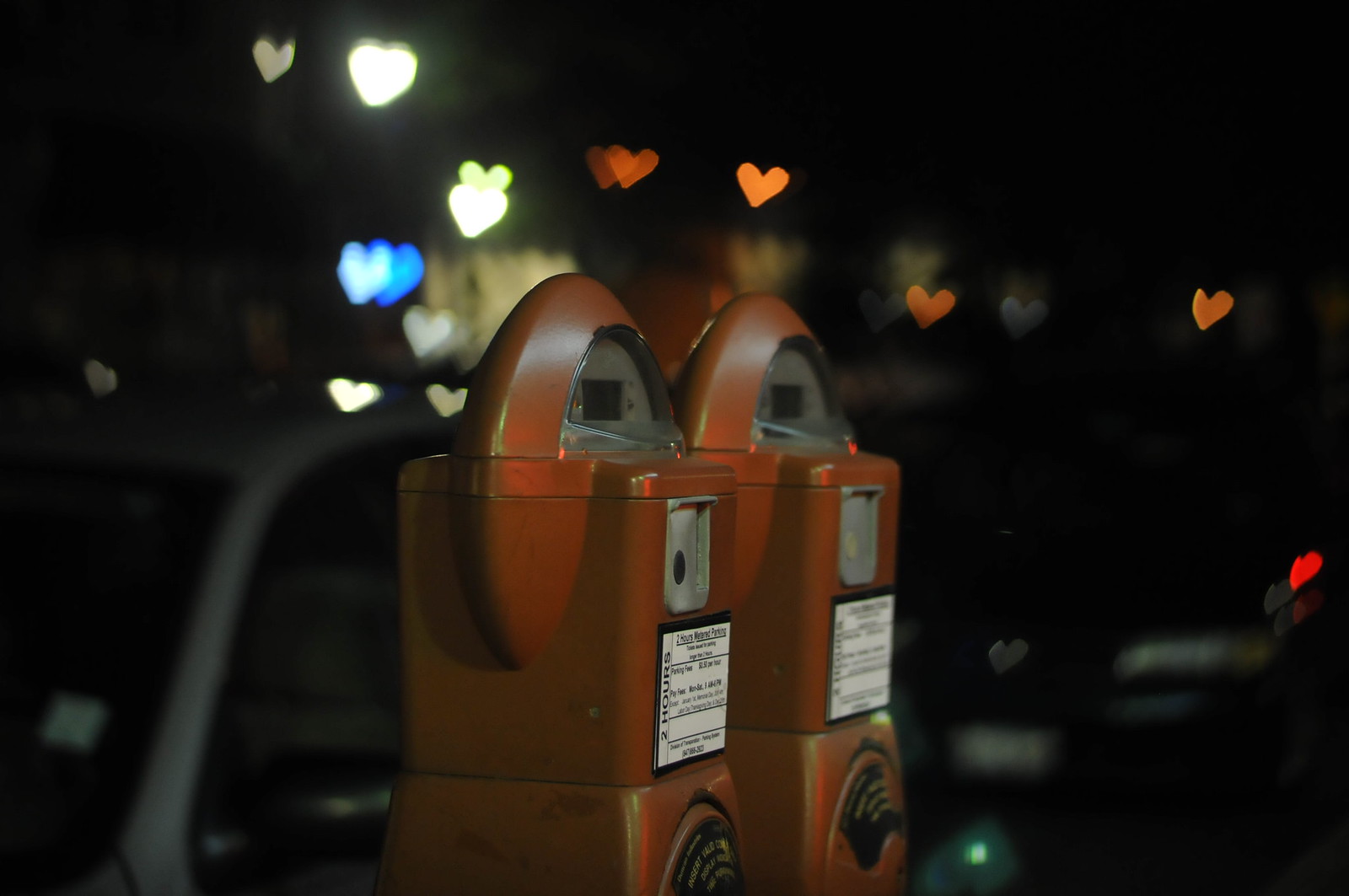This color photograph was taken at nighttime, capturing a scene centered on two old-fashioned parking meters prominently positioned in the middle of the image. The meters, which appear as a brownish rust color, exhibit a distinctive square base and an arched top, with a glass display on the front, possibly showing numbers. A silver component just below the display seems designed for coin insertion, and there's a black dial situated towards the bottom, giving it an antiquated look. The meters are positioned at an angle, facing towards the right, and are illuminated by artificial light, making them stand out sharply against the dark backdrop.

In the blurred background, a white car is partially visible on the left, with its top frame, side windows, windshield, and hood discernible. Adding a whimsical touch to the scene, multiple heart-shaped lights in shades of red, orange, blue, and white are scattered across the upper and central parts of the image, seemingly floating in the dark sky, suggesting a night filled with romantic or artistic lighting effects. A black vehicle is faintly visible in the bottom right corner, enhancing the nighttime urban atmosphere. The stark contrast between the sharply focused parking meters and the softly blurred surroundings, including the heart lights, creates a striking and evocative nighttime street scene.